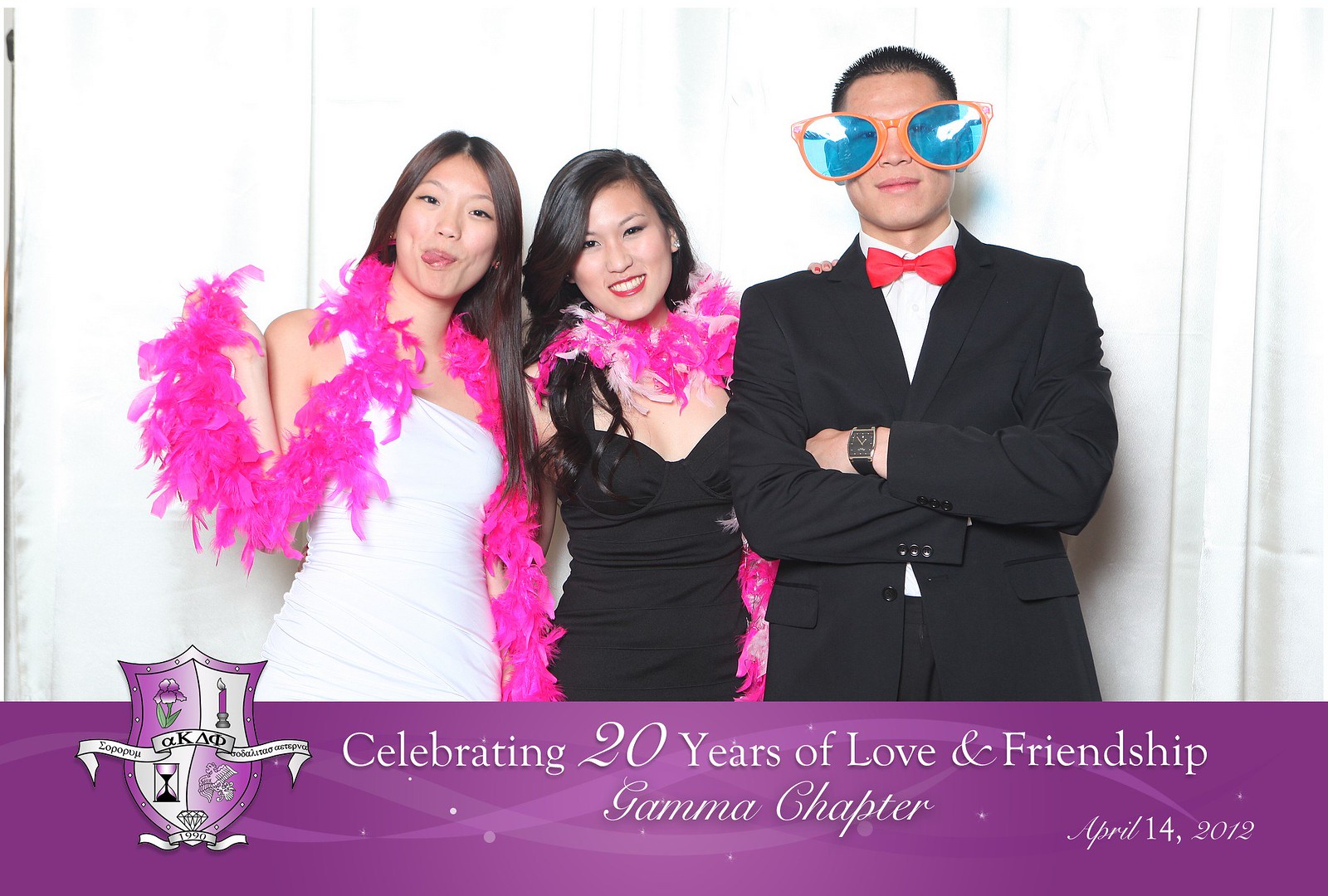In this image, three Asian individuals are posed against white curtains, creating a festive and celebratory atmosphere. From left to right, the first person is a dark brown-haired woman dressed in a white one-shoulder dress, adorned with a pink feather boa around her neck. Next, in the middle, stands a black-haired woman in a black strapless dress, also wearing a pink feather boa. To the right is a black-haired man dressed in a sophisticated black suit, a white dress shirt, a red bow tie, and a black wristwatch. He adds a touch of humor to the scene with his comically large clown sunglasses, featuring an orange frame and blue-tinted lenses. A magenta banner at the bottom of the image reads, "Celebrating 20 Years of Love and Friendship, Gamma Chapter, April 14, 2012," alongside the Greek letters representing the sorority or fraternity's logo.